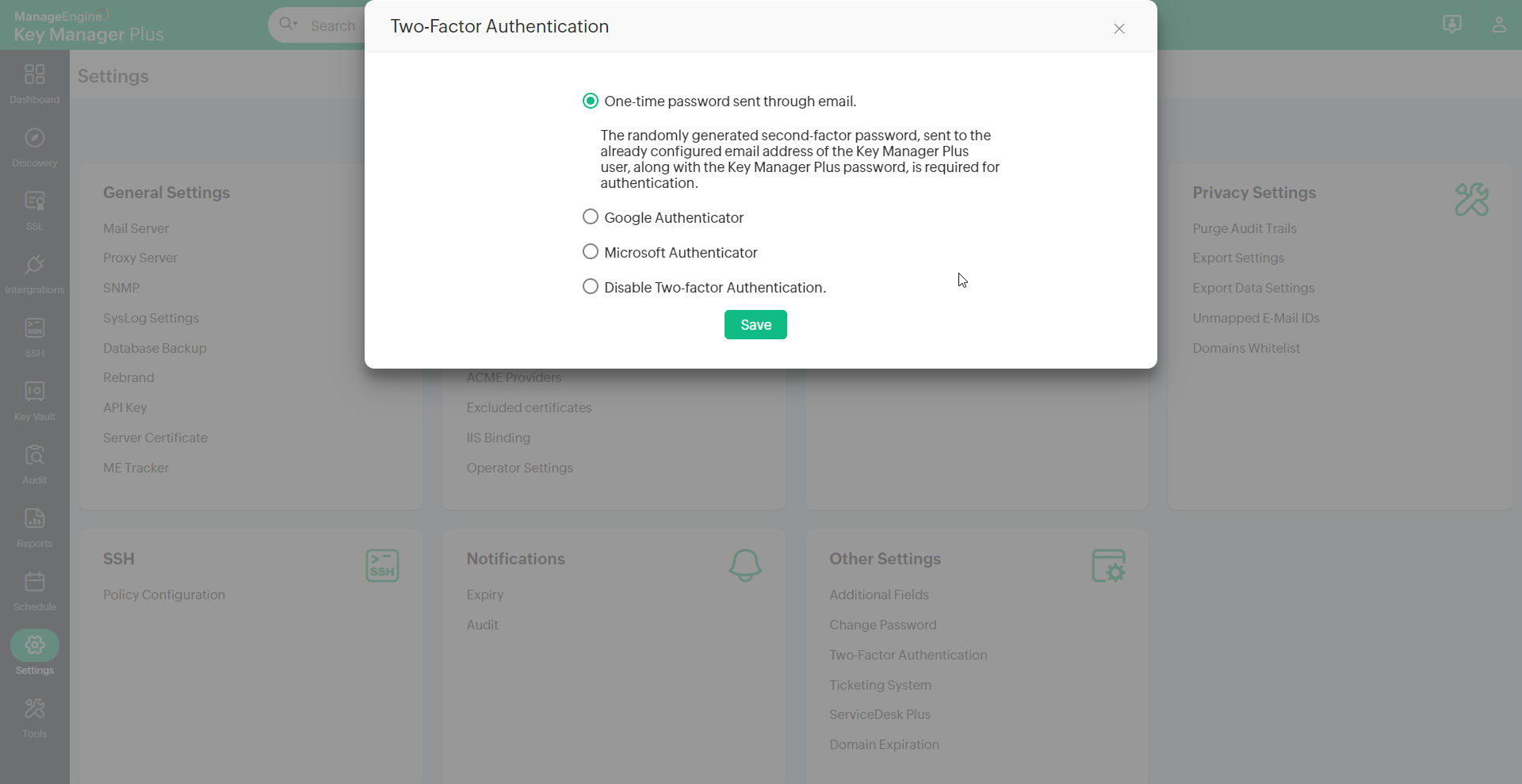The image showcases the interface of Key Manager Plus, a component of ManageEngine, specifically within the Settings section. The vertical sidebar on the left side of the screen features various navigation buttons including Dashboard (represented by a house icon), Discover SSH (showing key icons hinting at encryption functionality), SSL, Keystore, Audit, Report, Schedule, Settings (which is highlighted in green), and Tools.

When Settings is selected, a detailed submenu appears on the right, listing options such as User Management, General Settings, Privacy Settings, SSH, SSL, Notification, Additional Fields, Change Passwords, Two-Factor Authentication, Ticketing System, Service Desk Plus, and Domain Exploration. The interface currently focuses on the Two-Factor Authentication settings.

In the Two-Factor Authentication settings, at the top, an option for "One-time password sent through email" is selected, with a blue bubble highlighting the choice. This setting describes that a randomly generated second-factor password will be sent to the predetermined email address of the Key Manager Plus user. Other options within this section include using Google Authenticator, Microsoft Authenticator, or disabling Two-Factor Authentication entirely. At the bottom of this section, there is a green "Save" button to apply any changes made.

In the top-right corner of the interface, adjacent to the search bar, there are icons for initiating text communication (resembling a comment bubble) and accessing admin functions.